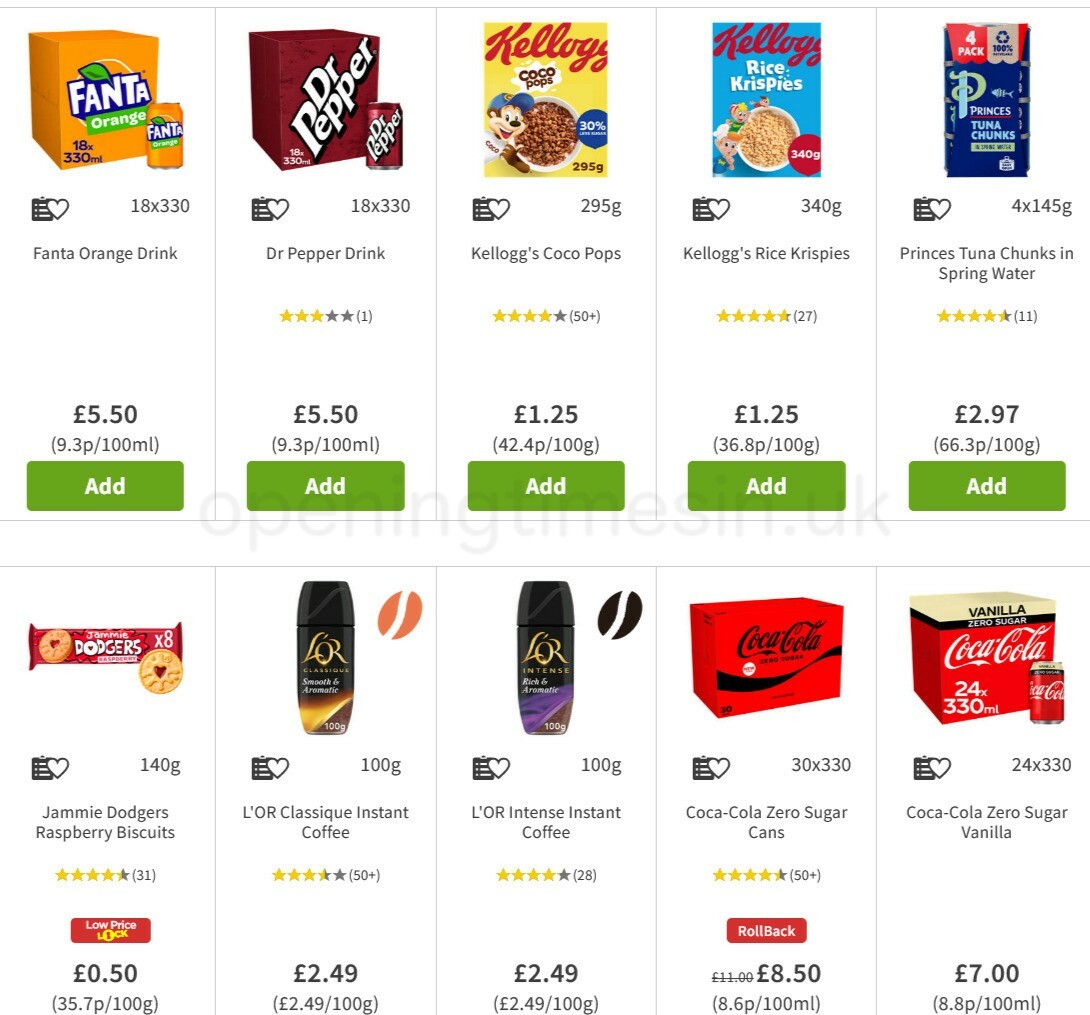This webpage displays a vibrant collection of various items, each neatly categorized within distinct boxes, separated by black lines both horizontally and vertically. Here's a detailed breakdown of the items featured:

1. **Fanta Orange Drink:**
   - **Description:** The box is adorned in orange, featuring the Fanta logo in white with a blue outline and a green leaf with light and dark green shades giving it a 3D effect. Below this, a green rectangle states "orange" in white.
   - **Details:** "18X 330ml" is noted in bold blue on the left, accompanied by an image of an orange cylindrical Fanta can displaying the same logo. Beneath this, similar to a clipboard icon with a heart (possibly for list creation), it describes the "Fanta orange drink."
   - **Price:** €5.50, with a cost breakdown of 9.3p per 100ml. 
   - **Button:** An add button is available for selection.

2. **Dr. Pepper:**
   - **Description:** Similar in structure to the Fanta box, it showcases a black background with the Dr. Pepper logo in white, and "18X 330ml" labeled similarly.
   - **Details:** The central section displays a single review, rating it 3 out of 5.
   - **Price:** €5.50.
   - **Button:** An add button is provided.

3. **Kellogg's Cocoa Puffs:**
   - **Description:** The image cuts off the right side of the red "Kellogg's" logo. It features a chipmunk clad in a blue hat with a red "C", a yellow background, and a white t-shirt with "cocoa" written in brown.
   - **Details:** Dark brown Cocoa Puffs, with some tan and light brown pieces, are depicted. A blue bubble states "30%" in white amidst other unreadable white text.
   - **Size:** 295g.
   - **Rating:** 3.9 out of 5 from over 50 reviews.
   - **Price:** $1.25 (42.4p per 100g).
   - **Button:** An add button is included.

4. **Kellogg's Rice Krispies:**
   - **Description:** The dark red "Kellogg's" logo appears atop "Rice Krispies" in white. Iconic Rice Krispies characters are shown beside a bowl of tan and light brown Krispies.
   - **Details:** A balloon-shaped bubble indicates "340g" in white.
   - **Rating:** 4.7 out of 5 from 27 reviews.
   - **Price:** $1.25 (36.8p per 100g).
   - **Button:** An add button is available.

5. **Princes Tuna Chunks:**
   - **Description:** A dark blue box reads "Tuna Chunks" in white. Above this, a bold white "PRINCES" is set in a red, cloud-like rectangle. It mentions "4PAC" in white and "100%" with a recycle symbol in tan.
   - **Details:** Described as "Princes tuna chunks in spring water".
   - **Rating:** 4.5 out of 5 across 11 reviews.
   - **Price:** €2.97 (66.3p per 100g).

6. **Jammie Dodgers Raspberry Biscuits:**
   - **Description:** A red rectangular container wrapped in red plastic features a heart-shaped cookie with a red center, indicating jam or filling.
   - **Details:** Marked "8X" in white, the packaging reads "Jammie Dodgers raspberry biscuits." 
   - **Size:** 140g.
   - **Rating:** 4.3-4.2 out of 5 from 31 reviews.
   - **Price:** €0.50 (35.7p per 100g).

7. **L'Oréal Instant Coffee (Classic):**
   - **Description:** The cylindrical black container is embellished with gold and brown bands. 
   - **Details:** Labeled "L'Oréal Classic instant coffee."
   - **Size:** 100g.
   - **Rating:** 3.5 out of 5 from over 50 reviews.
   - **Price:** €2.49 (€2.49 per 100g).

8. **L'Oréal Instant Coffee (Intense):**
   - **Description:** This variant features purple and brown bands.
   - **Details:** Labeled "L'Oréal Intense instant coffee."
   - **Rating:** 4 out of 5 from 28 reviews.
   - **Price:** €2.49 (€2.49 per 100g).

9. **Coca-Cola Zero Sugar:**
   - **Description:** The red box with a black band accents the "Coca-Cola" logo and "zero sugar" label. 
   - **Details:** Located in the lower right, it indicates "30X 330ml".
   - **Rating:** 4.5 out of 5 from over 50 reviews.
   - **Price:** Originally €11, now €8.50 (8.60p per 100ml). 
   - **Feature:** A rollback price label in black and white.

10. **Coca-Cola Zero Sugar Vanilla:**
    - **Description:** Similar to the Zero Sugar variant but with a vanilla-colored band.
    - **Details:** "24X 330ml" is labeled.
    - **Rating:** Not explicitly mentioned.
    - **Price:** €7 (8.80p per 100ml).

Each product is well-presented with detailed descriptions, images, prices, and ratings, making the webpage user-friendly and informative for potential buyers.